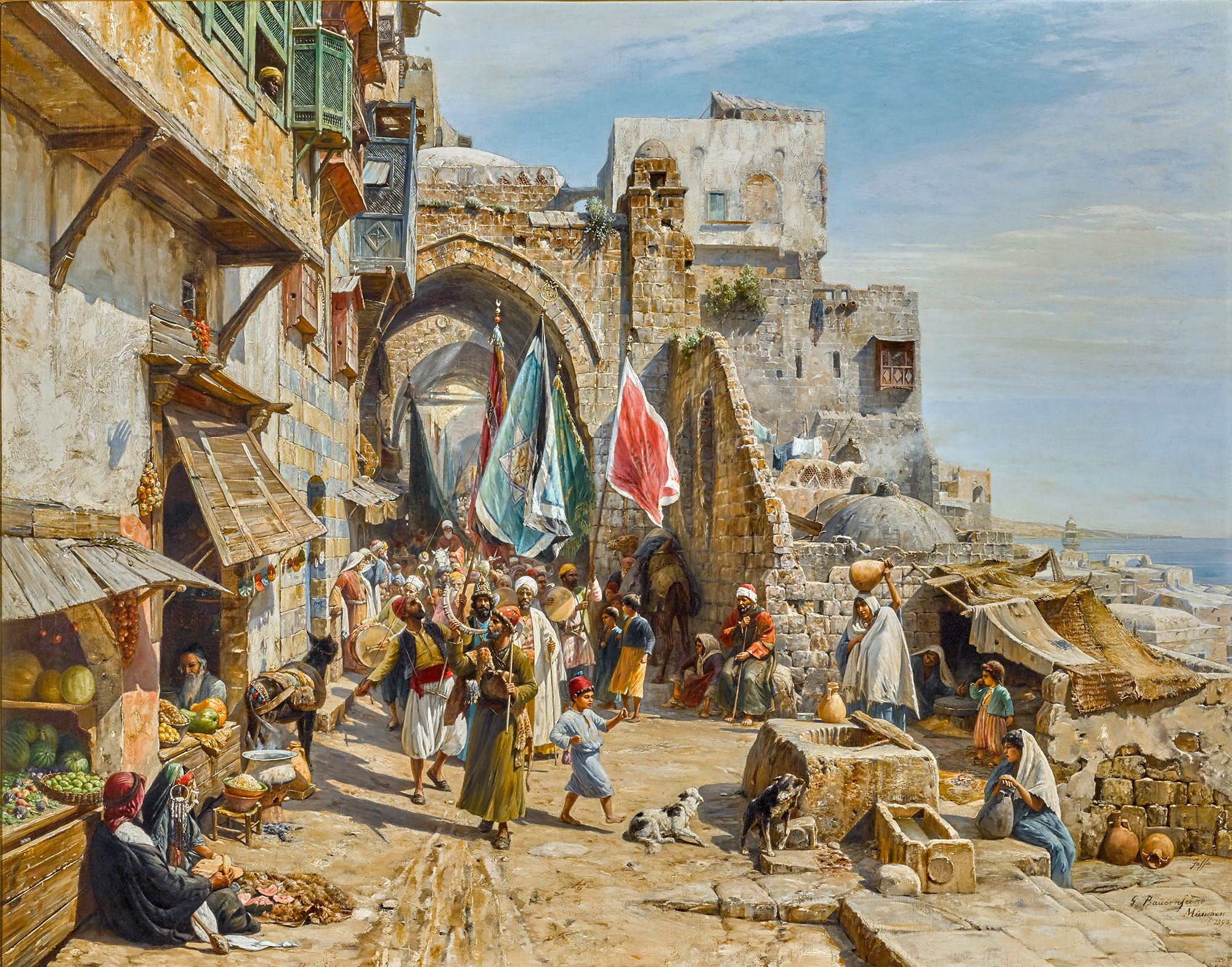This vibrant painting likely set in the 15th or 16th century captures an ancient festival unfolding in a bustling market town near the sea. At the center of this lively scene, a parade processes through an old, slightly dilapidated street, featuring flag bearers with blue-red flags, dressed in traditional garb with headdresses and robes. The lead figure stands out in a gold robe. 

To the left, a row of market stands offers fruits, with one proprietor seated attentively. Numerous figures populate the scene: women working with pottery, children playing, men playing instruments, and several shopkeepers tending to their wares, which include vegetables and cooking utensils. Animals such as dogs and a donkey also make an appearance.

The backdrop features a crumbling stone building with multiple floors, windows from which residents observe the parade, and an imposing brown archway from which the procession emerges. To the right lies the serene blue water, under a clear blue sky with white clouds. Despite the evident wear of the buildings and the slightly muddy ground, the townspeople—men, women, and children alike—seem engaged and spirited, offering a snapshot of community vibrancy during a historic celebration.